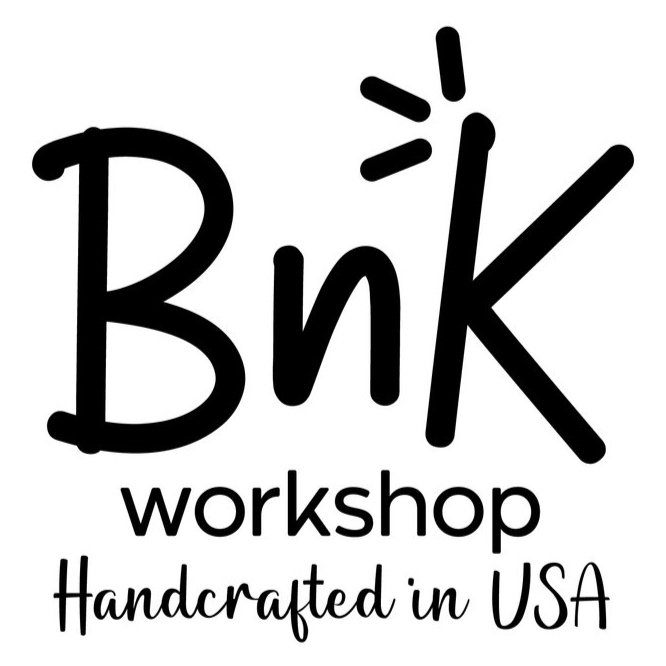The image is a simple, monochromatic logo for a business. It features bold, black letters on a white background. At the top center, there are large letters "B", "N" (in lowercase), and "K" in a handwritten-style font that looks as if it was drawn with a thick marker. The unique aspect of the "K" is that it has three small lines radiating from the top left tip, resembling sun rays or sparks. Beneath these letters, the word "Workshop" is displayed in plain, block lowercase letters. At the bottom, the phrase "Handcrafted in the USA" is written in a cursive font, emphasizing the artisanal and American-made quality of the products. The overall design is clean and straightforward, suggesting a proud, handcrafted ethos behind the brand B&K Workshop.